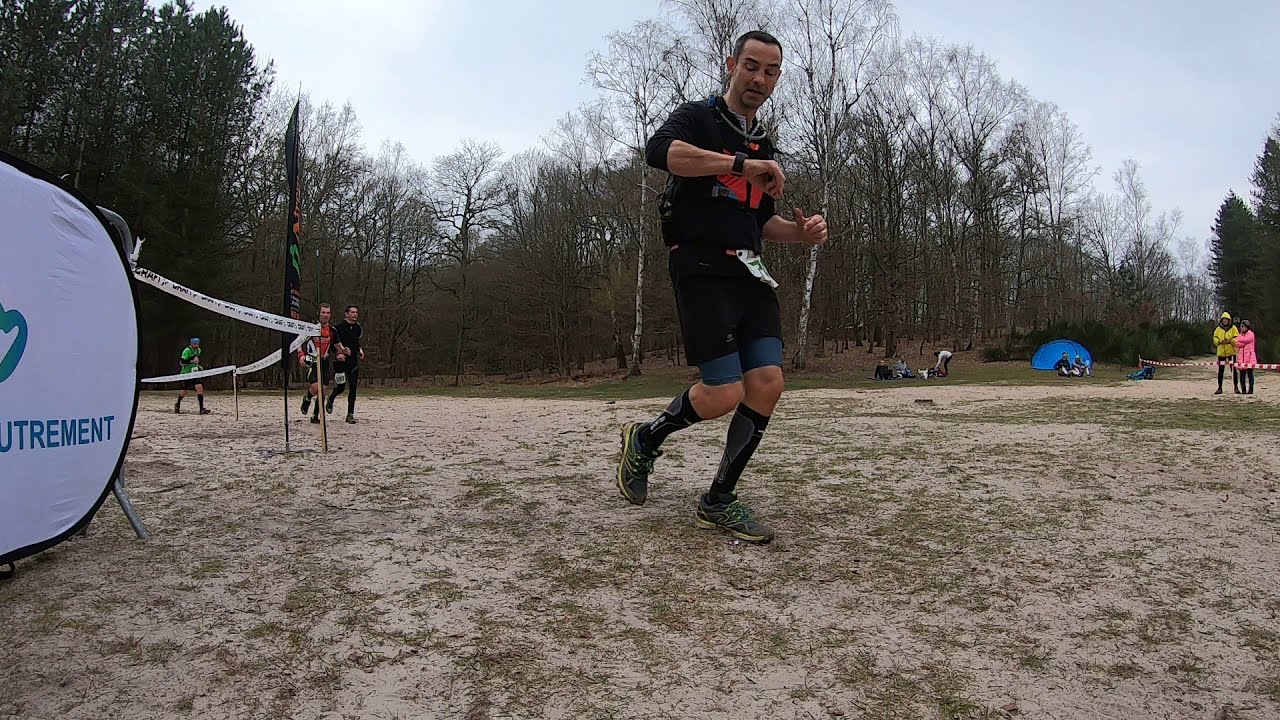In the center of the image, a man with dark, short hair and a thin build is running on a sandy, grassy terrain, possibly participating in a marathon or race. He wears a black top with a red print, blue biker shorts with black shorts over them, long black socks with a design, and gray shoes with green accents. A paper race number is attached around his waist, and he is checking a watch, likely a smart watch, as he runs. Surrounding him, there are several tall, bare trees suggesting a fall setting, and the sky above is mostly gray and white. In the near distance, there are other runners, as well as people sitting on the grass, who appear to be spectators. Two noticeable spectators include a woman in a pink jacket and a man in a yellow jacket with a hood. The event is demarcated by white caution tape, indicating the race path. A blue tent and additional observers are visible in the background. The overall scene is set in the daytime, amidst a countryside atmosphere.